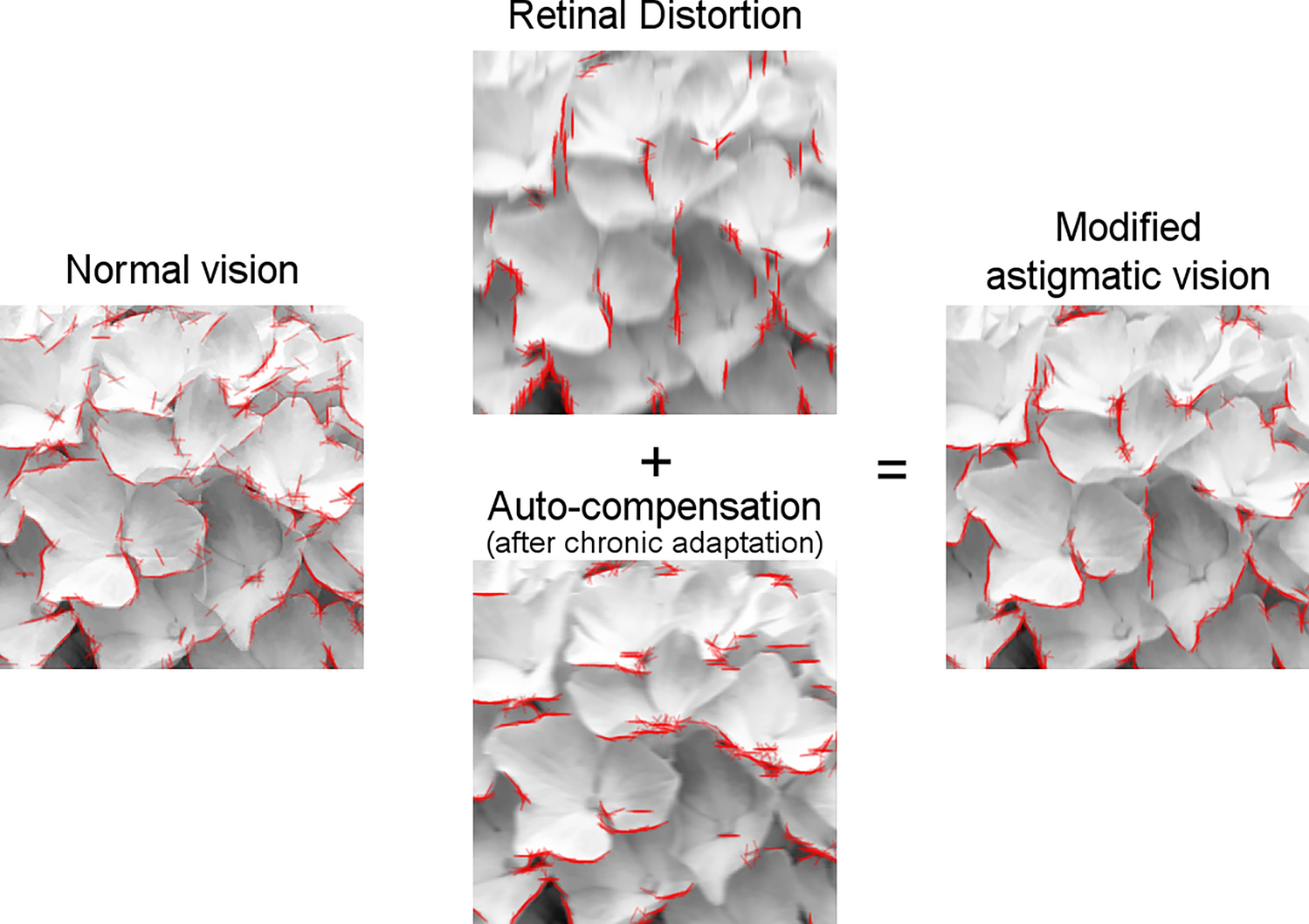The composite image features four square pictures set against a plain white background. Each picture contains a depiction of white flowers outlined with thin red lines. Starting from the left, the first picture is labeled "normal vision," showcasing a clear and focused view of the flowers. Moving to the middle, there are two vertically aligned images. The top middle image is labeled "retinal distortion" and presents a blurry version of the white flowers. Below it, the bottom middle image is described as "plus auto compensation after chronic adaptation," where the red outlines appear shifted, and the flowers remain somewhat blurry. The final image on the far right is labeled "equals modified astigmatic vision" and features the white flowers with a clearer, albeit still distorted, appearance. Black text is used for all the labels, with the overall layout providing a comparative study of different visual distortions.